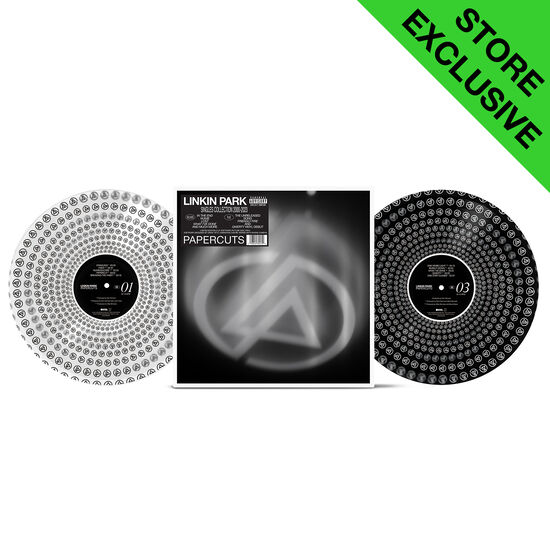This product image showcases a store-exclusive Linkin Park record set. In the upper right corner, a lime green triangle features the text "STORE EXCLUSIVE" in black, angled and prominent. The central focus is a Linkin Park album cover, which has a black background with an intricate circular logo that consists of overlays and patterns, including a central triangle design. Positioned on the upper left of this cover is a sticker that reads "Linkin Park" in white, above additional text, including the track title "Papercuts" and a barcode. Flanking the album cover are two vinyl records: the one on the left is a lighter shade, white with a black label and a circular pattern, while the one on the right is black with a similar design, the label in the middle marked "03."